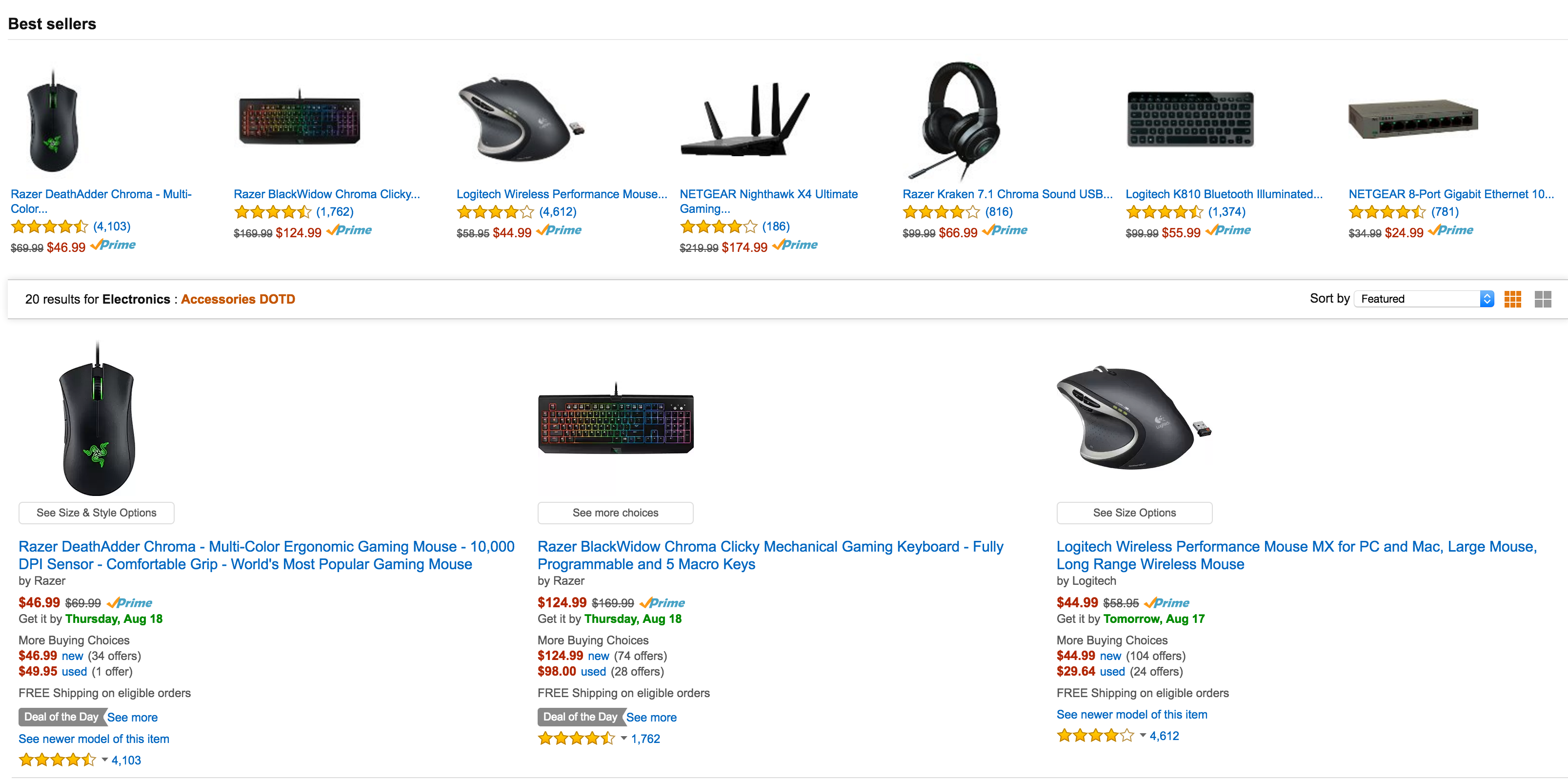This image appears to be a product page, potentially from an e-commerce site like Amazon, showcasing a selection of gaming and technology peripherals. At the top from left to right, the products featured include:

1. **Razer DeathAdder Chroma Multicolor Mouse** - A highly precise and customizable gaming mouse known for its ergonomic design and RGB lighting.
2. **Razer BlackWidow Chroma Click Keyboard** - A mechanical gaming keyboard renowned for its tactile and clicky keys, along with vibrant RGB backlighting.
3. **Logitech Performance Mouse** - A versatile and high-performance mouse suitable for both gaming and productivity.
4. **Nighthawk X4 Ultimate Gaming Router by NittoCore** - A robust wireless router designed to deliver superior gaming performance and minimal latency.
5. **Razer Kraken 7.1 Chroma USB Gaming Headset** - An immersive audio device offering 7.1 surround sound and customizable lighting.
6. **Logitech K810 Bluetooth Keyboard** - A sleek and portable keyboard featuring Bluetooth connectivity, ideal for multiple devices.
7. **Netgear 8-port Gigabit Ethernet Switch** - A reliable network switch providing high-speed Ethernet connectivity for up to 8 devices.

At the bottom, a zoomed-in view highlights the first three products from the top row:
- The **Razer DeathAdder Chroma Mouse**,
- The **Razer BlackWidow Chroma Keyboard**,
- The **Logitech Performance Mouse**.

This detailed layout showcases the premium features and design elements of each product, catering to gamers and tech enthusiasts.